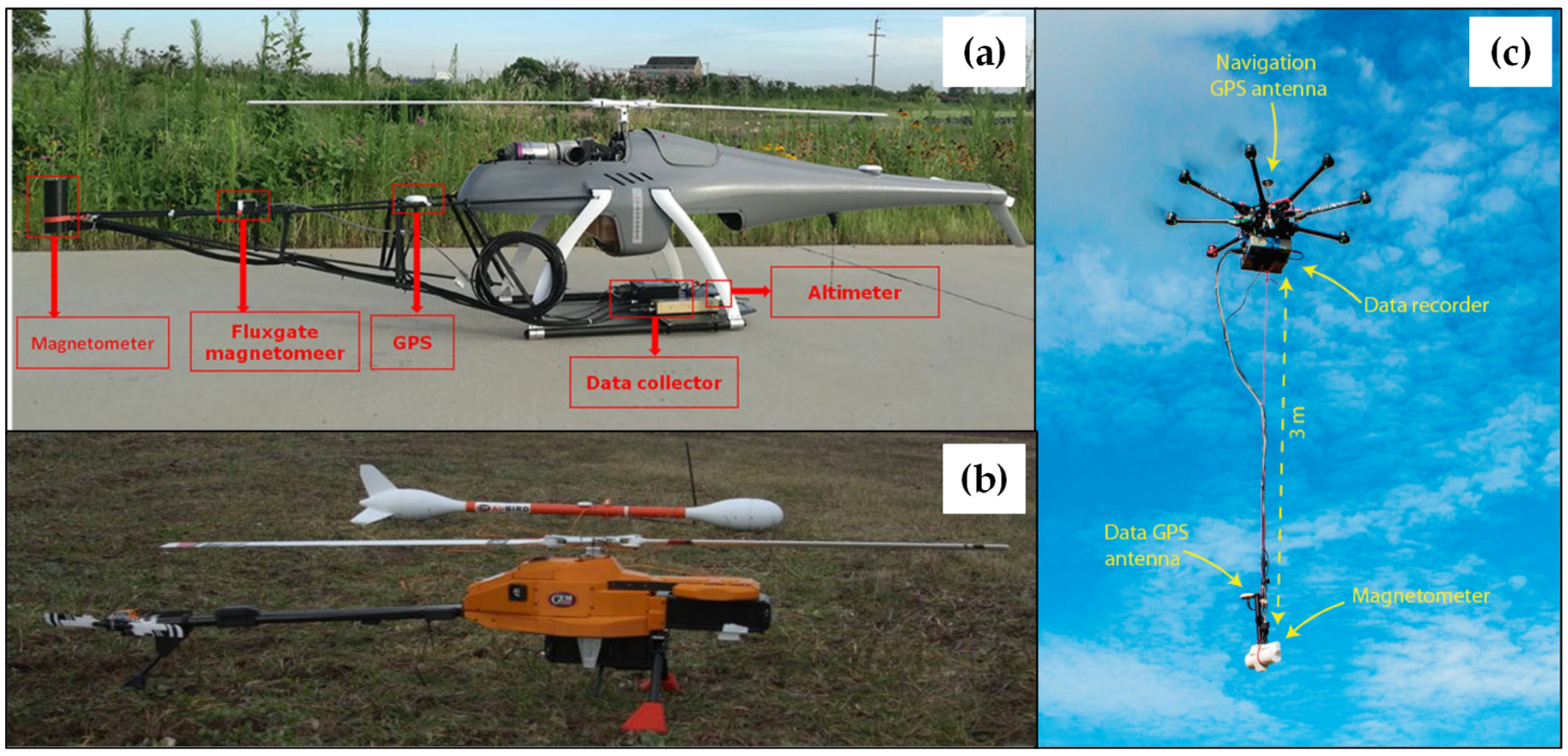The image showcases three distinct photographs labeled A, B, and C. 

**In Photograph A,** located at the top left, a small gray remote-controlled helicopter is shown resting on a concrete ground against a backdrop of a green field. The details of the helicopter are labeled with red description boxes. From left to right, these labels include: Magnetometer on the tail, Flux Gate Magnetometer, GPS, Data Collector near the center, and Altimeter. 

**Photograph B,** positioned at the bottom left, features a small orange helicopter with a white torpedo-like structure above its rotors, sitting on grass. 

**Photograph C,** on the right, depicts a drone flying against a bright blue sky with sporadic clouds. The drone has a navigation GPS antenna at the top, a square data recorder with several protruding diodes arranged in a circular pattern, a GPS antenna, and a magnetometer at the bottom, connected by a wire extending approximately three meters down.